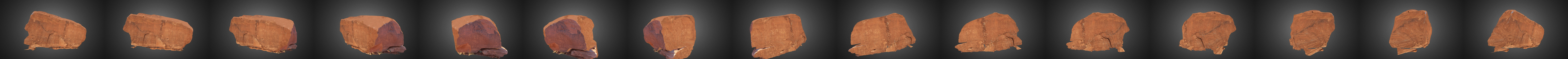The image depicts a long, thin, horizontal black bar, approximately one inch high, against a white background. Along this bar, there are 15 spaced objects that resemble rust-colored rocks, varying in shape and orientation. Each rock appears to be encompassed by a subtle blue circular smudge, giving the illusion of a transparent or translucent layer around them. The bar itself is divided into multiple squares, each hosting one rock in its unique configuration. The overall presentation suggests a design where each segment highlights a distinct rust-tan rock, positioned over a barely noticeable blue backdrop, maintaining uniformity in their spacing along the black stripe.